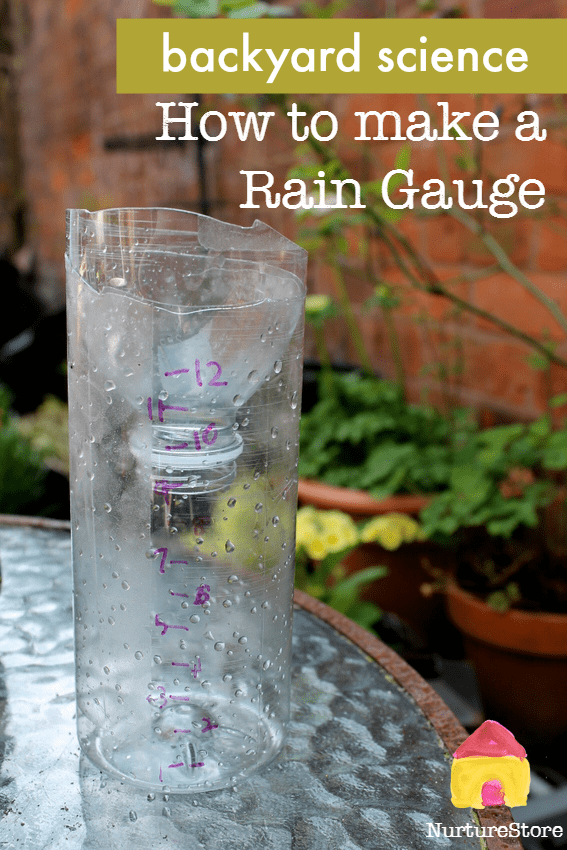The photograph, designed as a poster image for a blog titled "Backyard Science: How to Make a Rain Gauge," features a kid-style painting of a small house with the text "Nurture Store" in the bottom right corner. The central focus of the image is a homemade rain gauge created using a one-liter plastic bottle, which has been cut in half. The top half of the bottle is inverted to function as a funnel, and purple marker lines are drawn on the side, marking measurements from 1 to 12 inches. The rain gauge is positioned on a wavy glass patio table with a brown rim. In the background, there is a brick fence wall adorned with large ceramic pots filled with various plants and flowers. The overall dimensions of the image are approximately four inches wide by seven inches tall, and the text "Backyard Science" appears in a horizontal dark yellow bar at the top right, followed by "How to Make a Rain Gauge" in white font below it.